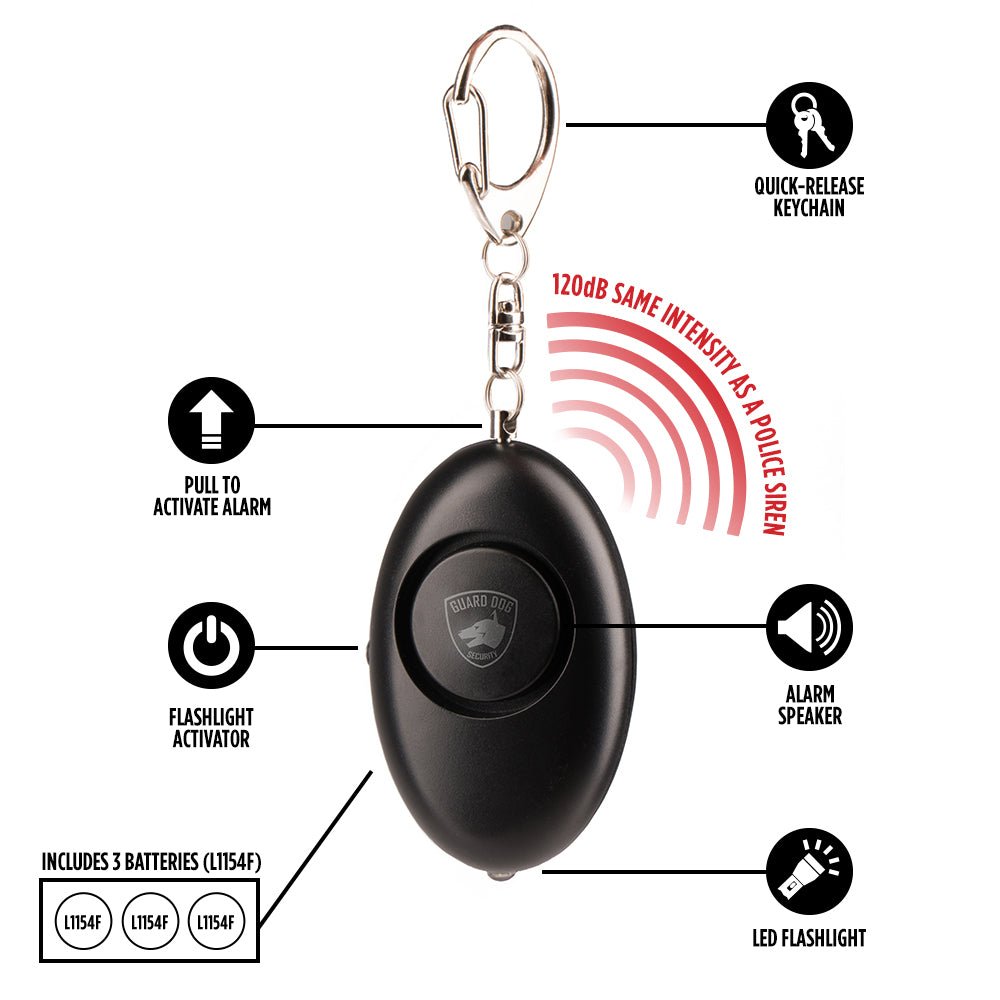This image features a detailed product diagram of a quick release keychain alarm system on a white background. The central element is a black, handheld, egg-shaped alarm device with a circular button in the middle bearing a white logo that reads "Guard Dog Security," accompanied by a dog head icon. Attached to the top of the alarm is a silver chain resembling a carabiner, connected via a jump ring.

On the left side of the image, a line points to the chain and is labeled "Pull to Activate Alarm," with an upward arrow for emphasis. Below it, another label reads "Flashlight Activator," followed by a note that the package "Includes Three Batteries" (specified as L1154F in a small rectangular diagram showing three circles).

On the right side, there's a red, arching, rainbow-like wave symbol labeled "120 dB, same intensity as a police siren." Further down, additional captions indicate the functionalities of the device: "Alarm Speaker" with a speaker icon and "LED Flashlight" with a flashlight icon. The overall diagram clearly labels each component and feature of the keychain alarm, highlighting its quick release mechanism, powerful alarm sound, and built-in flashlight.